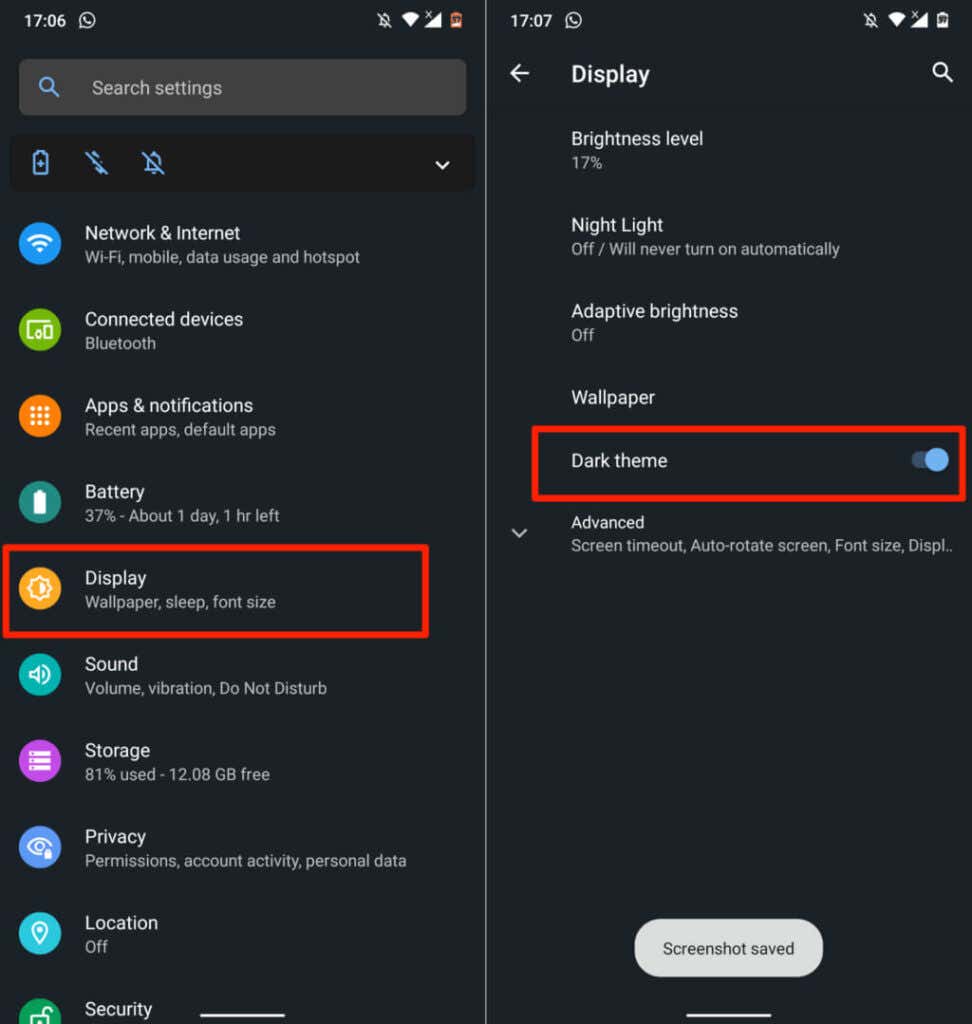The image is divided into two sections, reflecting the settings menu of a smartphone, displayed in dark mode. The background is predominantly black, enhancing the visibility of the icons and text.

**Left Image:**
- At the top is a search bar labeled "Search settings."
- Below the search bar is a drop-down menu featuring three blue icons: 
  - Better self icon
  - Mobile data icon
  - Silence icon
- Following this section are various settings categories:
  - **Network & Internet:** Includes Wi-Fi, mobile data usage, and hotspot, represented by a blue and white Wi-Fi icon.
  - **Connected Devices:** Features Bluetooth settings with a green icon illustrating connected devices.
  - **Apps & Notifications:** Contains options for recent apps and default apps, marked by an orange and white icon.
  - **Battery:** Displays 37% remaining with an estimated one day and one hour left, indicated by a green icon with a white battery.
  - **Display:** Includes settings for wallpaper, sleep mode, and phone size. This category is emphasized with a red outline rectangle, indicating the selection, and is represented by an orange and white icon.
  - **Sound:** Covers vibration, volume, and Do Not Disturb settings, shown with a green and white icon.
  - **Storage:** Shows 81% used with 12.08 GB free, illustrated by a purple and white icon.
  - **Privacy:** Includes payment and account activities, represented by an eye icon with a lock on a blue background.
  - **Location:** Indicates that location services are off, with a blue icon featuring a white location pin.

**Right Image:**
- Focuses on the "Display" settings. Below the "Display" heading, the following items are listed:
  - **Brightness Level:** Set at 17%.
  - **Night Light:** Off, with a note that it will never turn on automatically.
  - **Adaptive Brightness:** Currently off.
  - **Wallpaper**
  - **Dark Theme:** Highlighted by a red rectangle and showing that the toggle switch is on (blue).
- Below these options is a drop-down menu labeled "Advanced," which includes settings for screen timeout, auto-rotate screen, and phone size.
- At the bottom of the image, there is a pop-up notification stating "Screenshot saved."

The detailed caption provides an insightful view into the smartphone settings interface, showcasing various customizations available to the user, with particular emphasis on the Display settings and the active dark mode.